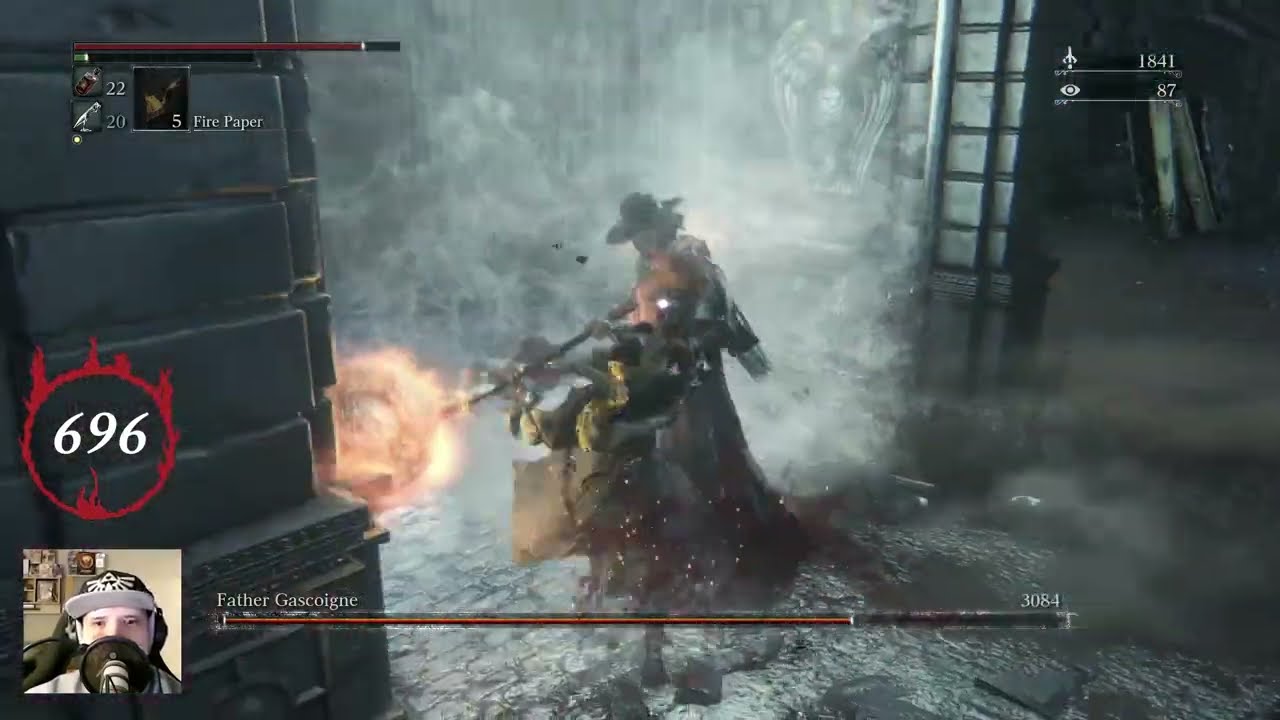The image depicts a webcast of a video game stream featuring a player in a black baseball cap seated in a gaming chair with a microphone partially obstructing his face. His eyes are visible, and the background of his room can be seen. The main game screen shows an intense battle scene framed by various game indicators. The focal point is a character in the center wearing a black cowboy hat and robes, identified as "Father Gascoigne" by the health bar underneath his figure, which is about 75% full. This character is wielding a staff-like weapon with a flamethrower emitting flames from the tip. There is another character in front of Father Gascoigne, engaging in combat, with blood spewing out.

The scene takes place in a foggy hallway featuring debris, smoke, and broken cobblestone, adding to the chaotic atmosphere. In the background, there is a vase with angel wings on either side and a pillar. The top left section of the screen provides details on the player's current status, including equipped weapons like "fire paper," ammo count, and other resources. A red circular logo with the number "696" is prominently displayed above the streamer’s thumbnail, which is positioned at the bottom left of the screen. The upper right corner also lists additional game indicators, such as a numeric value "3084" and a partly depleted red health bar, alongside a small black box with the number "22" and a white bird icon with the number "20."